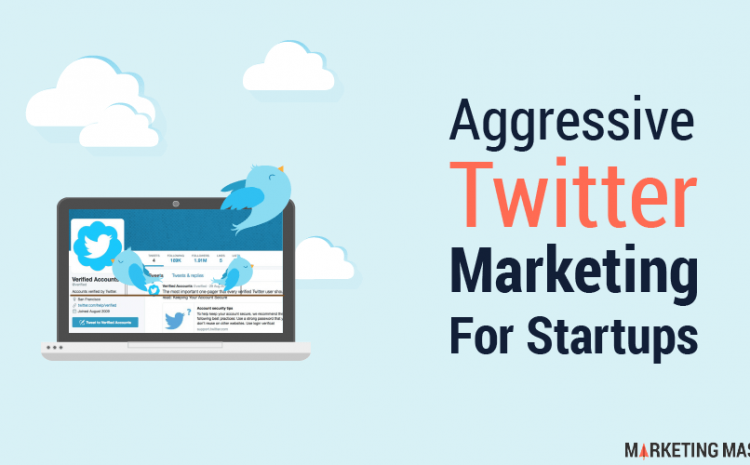This image is a screenshot of an advertisement designed to promote marketing services for startups on Twitter. The photo is in landscape orientation, with dimensions that are wider than they are tall. The background of the image is a light blue color, adorned with scattered clouds primarily positioned near the top left, center left, and middle left areas.

In the background, there is a cartoon illustration of a laptop. The laptop's frame is black, with a gray bottom edge. It features a light blue border running across the top of the screen, along with a prominent white Twitter bird icon encased in a blue border. Several other blue birds are superimposed onto the computer screen, emphasizing the Twitter branding.

The central part of the screen displays a white, rectangular box in landscape orientation, where the words "verified account" are visible. Below these words is a blue rectangular button with white text, which appears to be clickable, although the exact text is not legible.

To the right of the laptop screen, the word "aggressive" is written in black font. Underneath it, in larger orange font, the word "Twitter" is prominently displayed. Below that, in black font, the text "marketing for startups" is clearly visible. A watermark at the bottom of the image reads "marketing MAS," although it is partially cut off. The 'A' in "marketing" is stylized as an orange arrow or tent pointing upward.

Overall, the advertisement seems to be promoting a service aimed at helping startups with their Twitter marketing efforts.